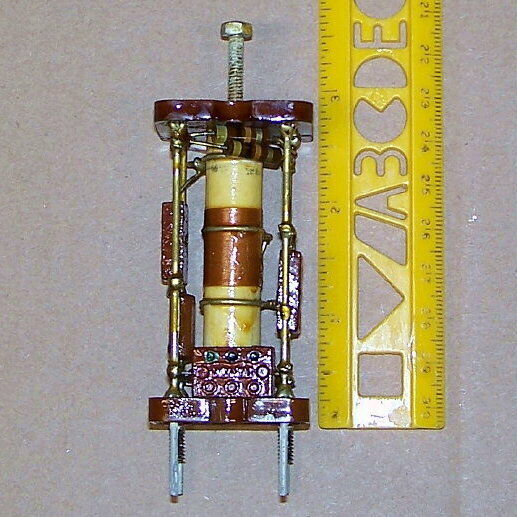The photograph showcases a cylindrical electric device prominently positioned on a flat, gray surface mottled with various brown spots. The device itself is characterized by a brown and beige cylindrical core, wrapped with brass-colored wires, set within a brass-colored frame painted with brown accents on both top and bottom. The cylinder runs vertically, flanked by four brass poles at each corner, reinforcing the frame's structure. Two bolts are visible, one at the top and one at the bottom, adding further stability.

To the right of the device lies a well-used yellow ruler, indicating that the device is approximately four inches long, excluding the additional length contributed by the bolts. The ruler’s inch measurements are positioned adjacent to the device, showing various black notches and numbers, while the centimeter markings extend off-screen. The ruler features cut-out stencils of geometric shapes and letters, such as squares, triangles, and the letter 'A', adding a unique touch to its worn appearance, evidenced by black paint chipping off the numerals.